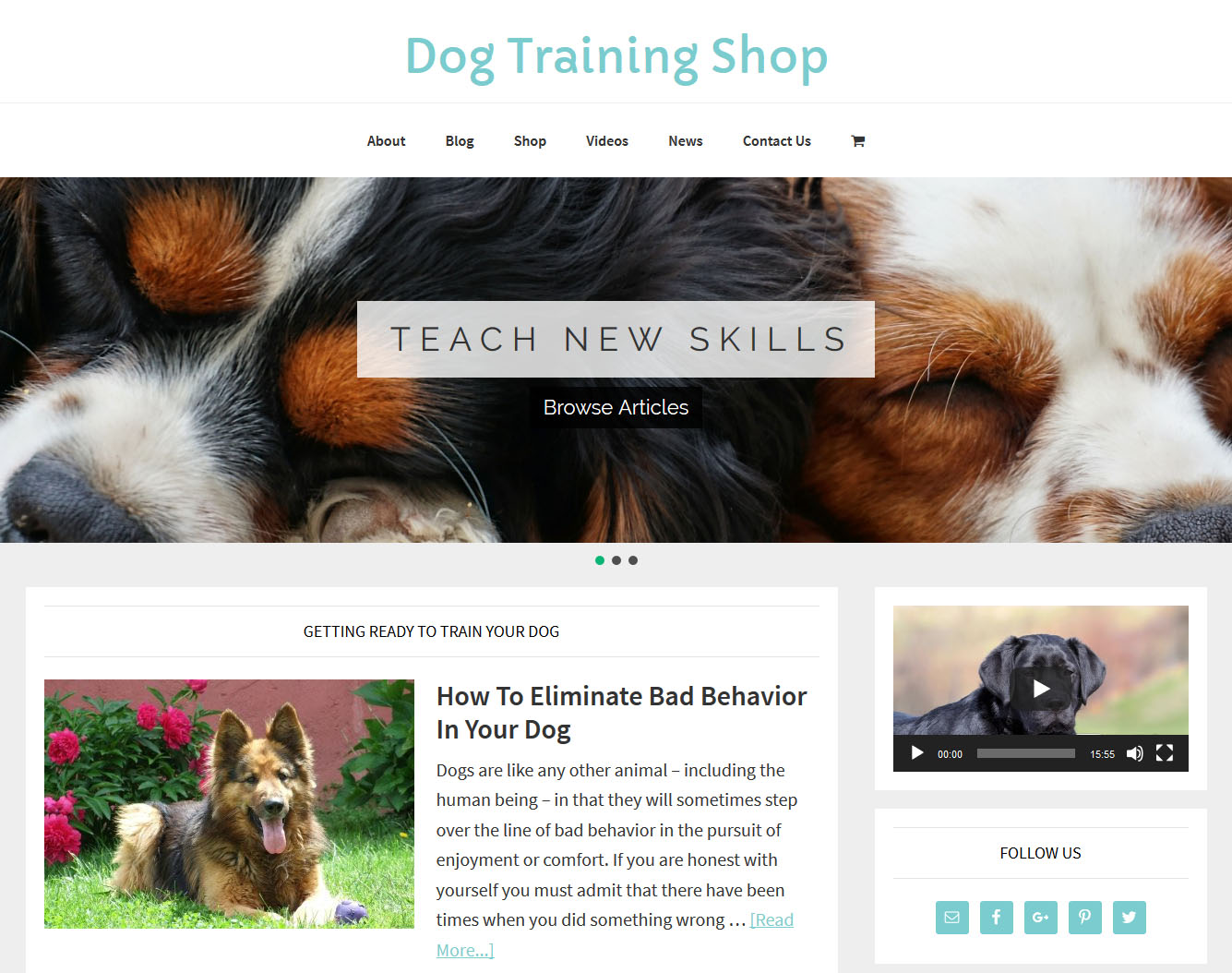A detailed screenshot of the "Dog Training Shop" webpage, featuring a green, curly text logo on a white background. Below the logo is a menu in smaller black text with options: About, Blog, Shop, Videos, News, Contact Us, and a shopping cart icon. Prominently displayed is a large banner image of two colorful dogs sleeping, one with predominantly black fur with orange and white accents, and the other mostly orange with white markings on the head and nose. Centered on the banner is the article title "Teach New Skills," followed by a link to browse articles. Below this is an article titled "How to Eliminate Bad Behavior in Your Dog," accompanied by a picture of a German Shepherd with perked ears, sitting on a lawn with pink flowers in the background, basking in sunlight. The beginning of the article text is visible but truncated, with a link to read more.